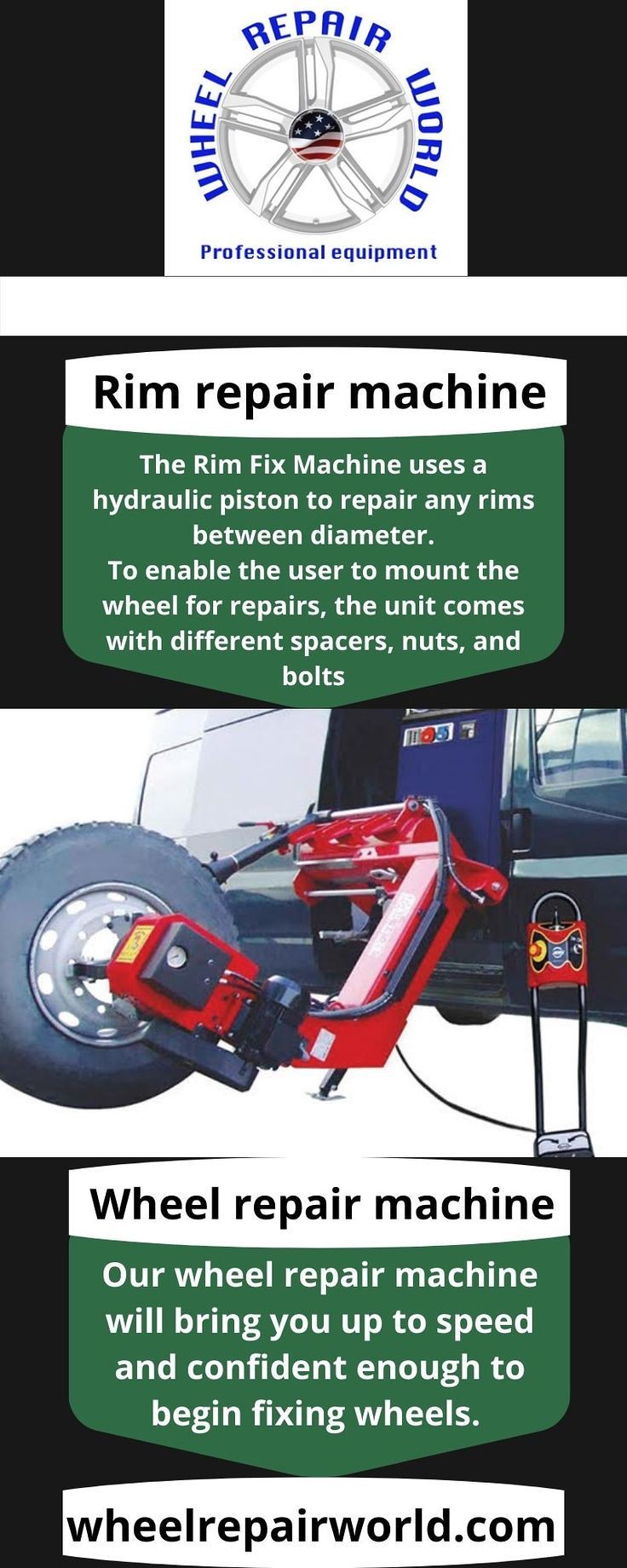The image is an advertisement for Wheel Repair World showcasing their professional equipment. At the top, in blue letters encircling a silver rim with an American flag in the center, it says "Wheel Repair World Professional Equipment" against a black background. Below, the text "Rim Repair Machine" appears in white against black, followed by another white text section on a green background detailing the Rim Fix Machine's capabilities: "The Rim Fix Machine uses a hydraulic piston to repair any rims between diameters. To enable the user to mount the wheel for repairs, the unit comes with different spacers, nuts, and bolts." There is a picture of the equipment, highlighting a red and black robotic arm mounted on a box-like structure, holding a wheel with a silver rim. The backdrop includes a van with a white stripe and a multi-colored post. Further down, another green box with white text promotes confidence: "Our Wheel Repair Machine will bring you up to speed and confident enough to begin fixing wheels," followed by the website "WheelRepairWorld.com" in black letters on a white background, all set against the same black backdrop. The image vividly presents the company’s high-tech wheel repair solution, emphasizing its efficiency and ease of use.